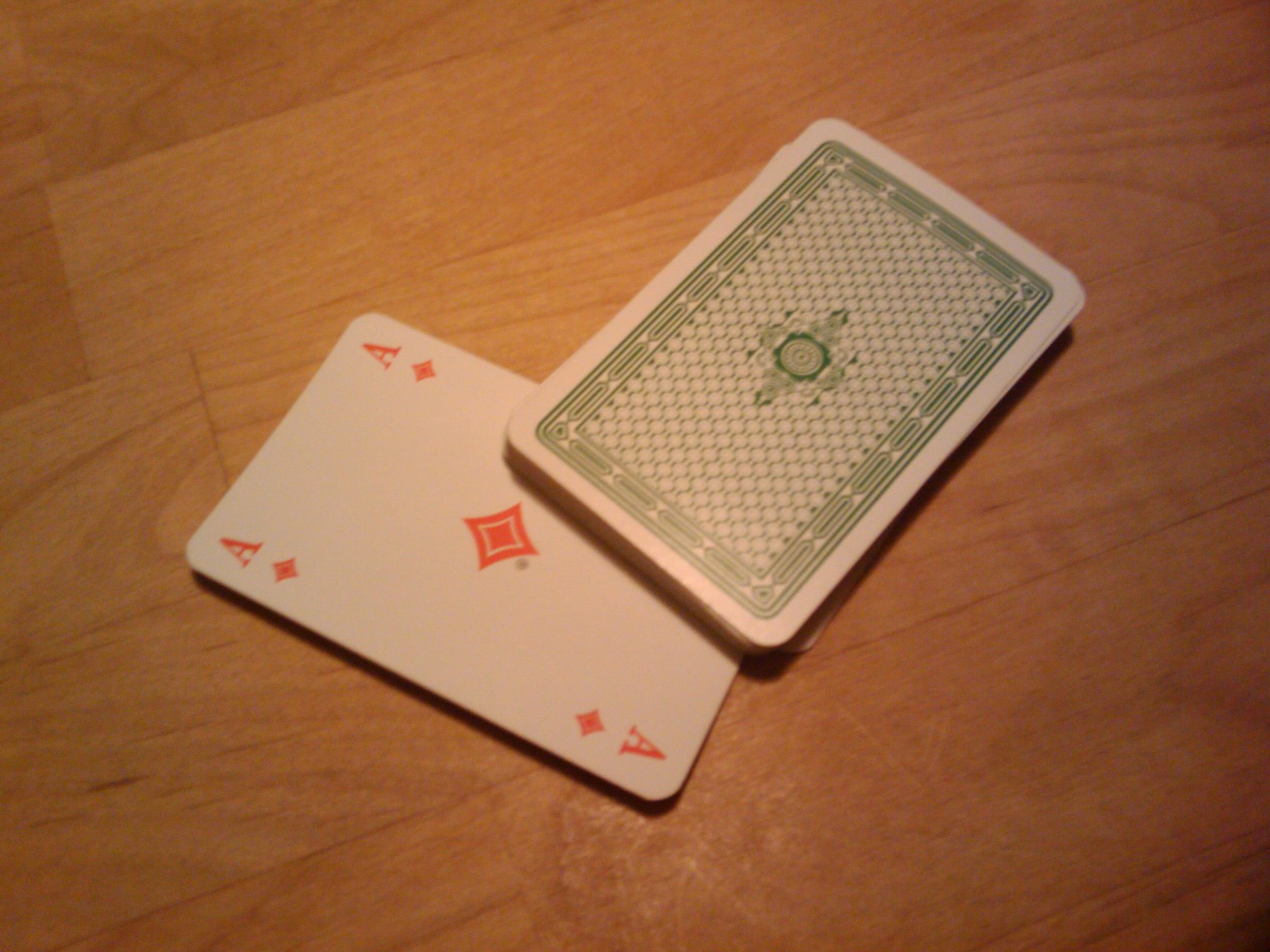The image features two playing cards positioned on a background that resembles a wooden floor, characterized by its caramel brown color and rectangular patterns. The top card has a white outer border, followed by a green-bordered frame with white accents. Within this green frame, there are multiple white circles grouped together, and at the center is a floral stamp. The card beneath, oriented in the opposite direction, is predominantly white and adorned with red 'A's located at the top right, top left, and bottom left corners. Just below each 'A' is a small red diamond shape. The central area of this card also features a larger red diamond shape. Both cards are meticulously positioned one overlapping the other, with the design of only one card fully visible.